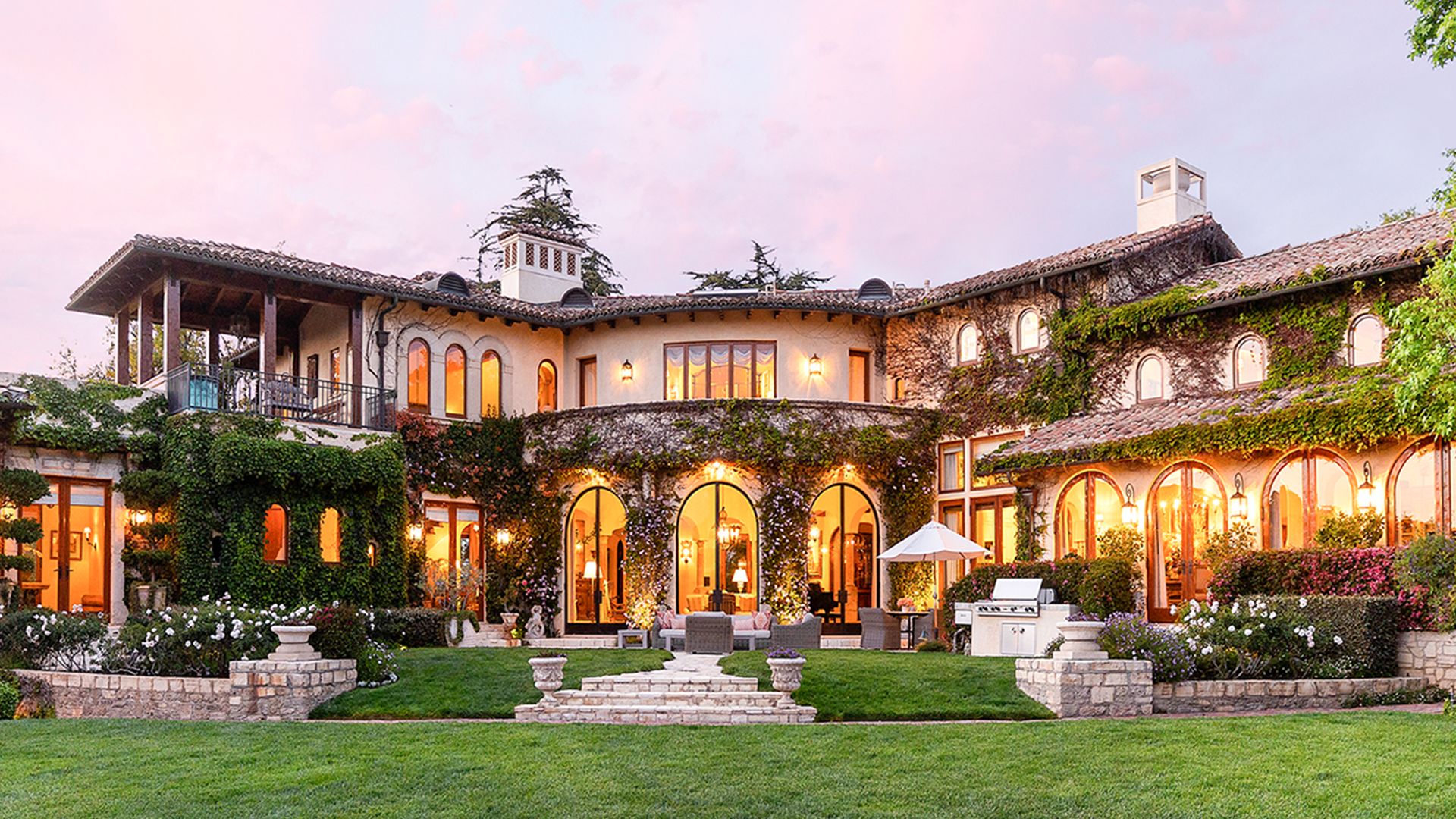This is a detailed, horizontally aligned rectangular 3D color rendering of a large two-story house, generated using an app such as SketchUp. The house is presented in a front elevation view, taken from a vantage point on the front lawn. The lush, green grass stretches from left to right at the bottom of the image. 

The house features a central round curve portion flanked by two extensions, one extending to the left and the other to the right. The central section includes three arched entryways leading up to a front porch with short stone steps. These steps are bordered by two decorative urns. Ivy plants cover the walls in this central area, enhancing the home’s elegant aesthetic.

The right section of the house showcases at least four arched windows on the lower level, with three smaller arched windows directly above them. Additionally, you can spot an outdoor grill and a patio area here. On the left side, the house boasts an upstairs balcony with a black railing, providing a spacious area for outdoor seating. Below this balcony, there is a small retaining wall adorned with an array of white flowers.

The house has a beige-colored tile roof, mostly covered in green moss, adding a rustic charm. There is also a white lookout structure on the top-right portion of the roof, and another white roof structure on the left center. 

The sky above is a picturesque blend of pinkish-white clouds and blue, indicating that the image was captured during the daytime. The overall style and setting of this image reflect a highly detailed and realistic 3D rendering of a beautiful home’s front facade.